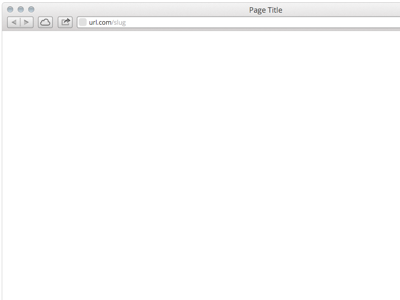In this screenshot of a web browser interface, the main area is blank, signifying either an empty page or a loading screen. At the top-left corner, there are three small circles typically representing window control buttons: close, minimize, and expand. Adjacent to these buttons, on the left side, are navigation buttons for forward and backward functions. Additionally, there's an icon resembling a cloud, potentially indicating sync status or cloud storage options.

Centered at the top is the address bar displaying the placeholder text "URL.com," with the text box having a light gray background. Next to the address bar, there's a small arrow icon indicating the capability to navigate backwards.

To the right of the address bar, the page title is displayed in dark gray text against a very light gray background, blending subtly into the interface. Contrasted against this are the expansive white areas that dominate the rest of the browser's visual. The overall aesthetic is minimalistic, emphasizing functionality and clean design.